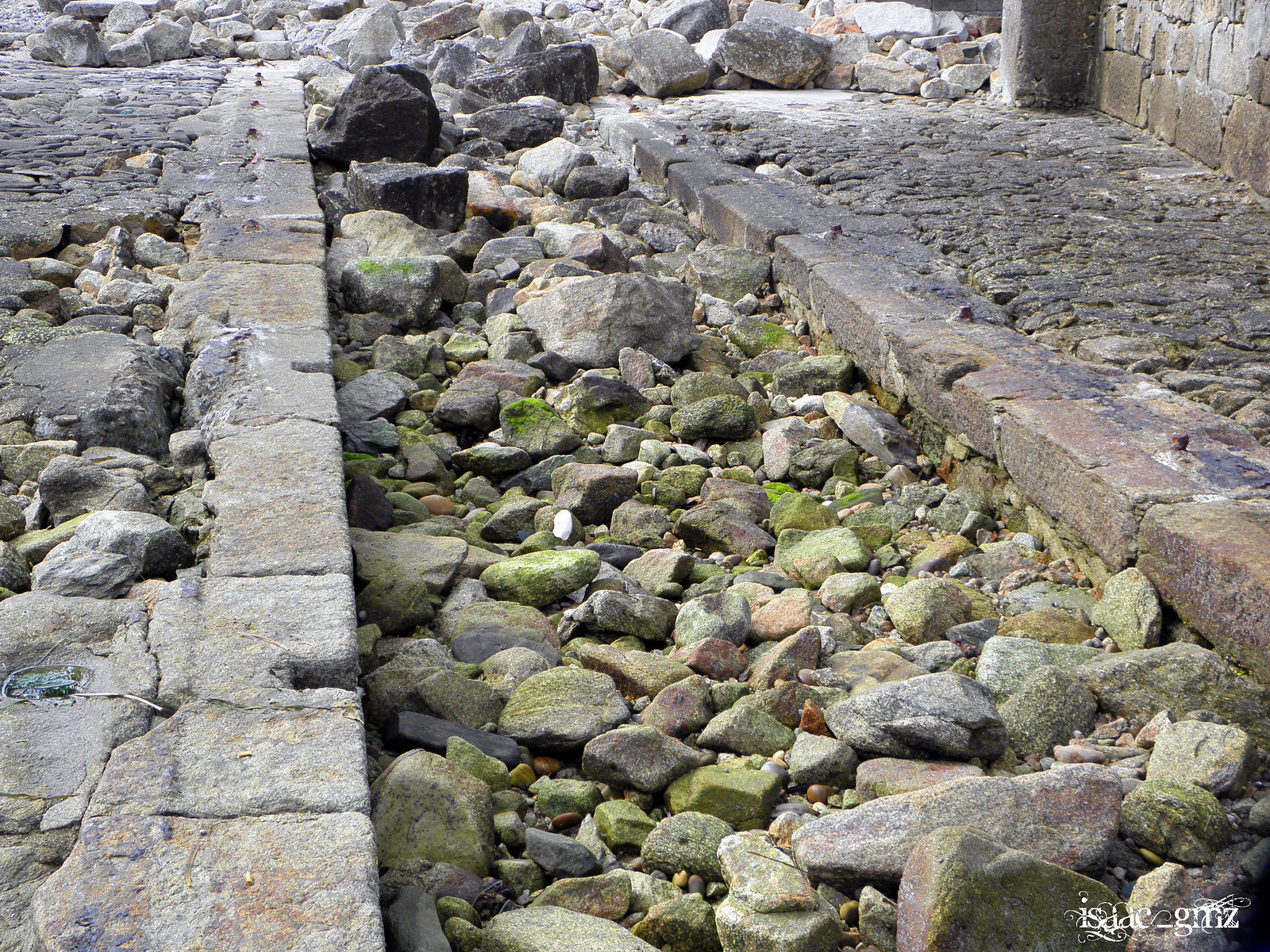The photograph captures an outdoor scene featuring a central channel filled with a variety of gray rocks and stones, ranging in size and many covered in patches of green moss. This rocky channel, which appears as if it once directed water flow, is flanked by two stone or brick pathways, reminiscent of ancient sidewalks or walkways. On the right side, the pathway seamlessly transitions into a stone wall, while the left side appears to be a less uniform repair using larger rocks. The setting has an air of antiquity, possibly an ancient structure or historical site, with the stones and pathways invoking the sense of a bygone era. Sunlight illuminates the area, highlighting the density of rocks that overflow from the channel and spread out onto the adjacent paths. At the bottom right of the image, white text reads "Isaac_GMZ," likely indicating the photographer’s watermark.